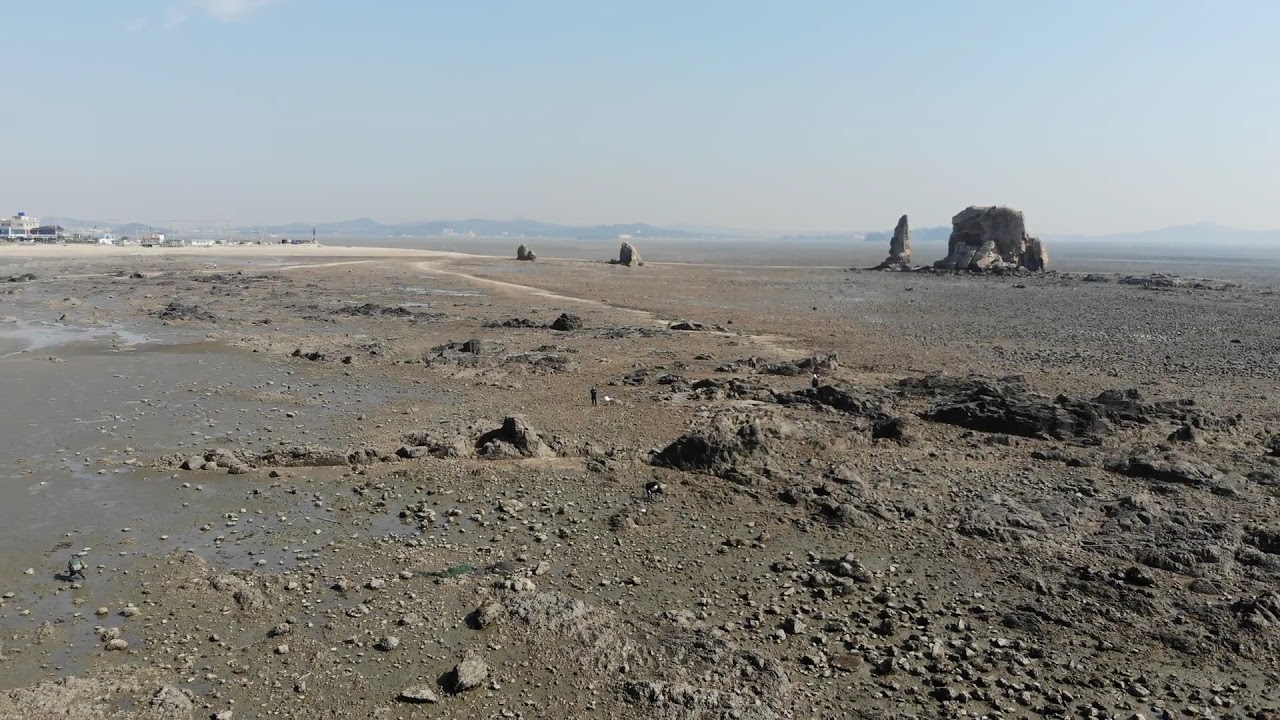In the foreground, there's a barren desert landscape with a muddy, dirt ground that appears recently rained on. The left side is particularly muddy, with some water pooling, and as you move right, low rocks protrude from the ground. The right side features prominent rock formations: a wide, flat-topped butte, and next to it, a narrow, Christmas tree-shaped butte. To their left are two smaller rock structures. In the upper left part of the image, some distant buildings are visible, connected by a dirt road. Beyond these structures, a row of blue-hued mountains stretches across the horizon under a mostly clear, slightly hazy sky, creating a desolate, almost lunar ambiance.